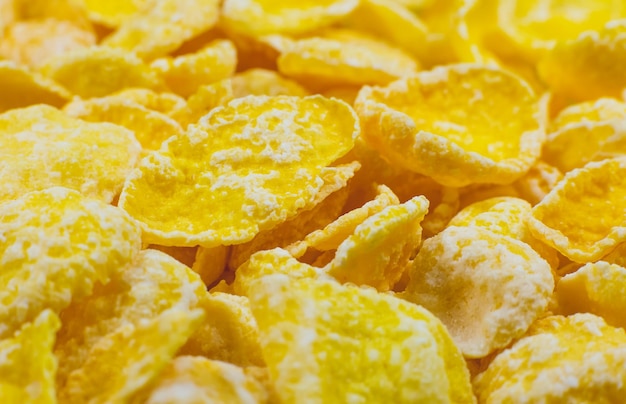This image is a small rectangular photograph, about 5 inches wide and 3 inches high, featuring a close-up of cornflakes or possibly frosted flakes. The flakes are predominantly yellowish-orange with irregular shapes and ragged edges, some of which are curled at the corners. Scattered among the flakes are areas with a white coating, possibly sugar. The clustering of flakes suggests they are in a bowl, viewed from a half-inch or an inch above. The lighting, which creates a reflection, potentially affects the color perception. The image's top portion is slightly blurred, contributing to an overall lack of sharpness. Notably, one flake in the bottom right corner is almost entirely coated in white.